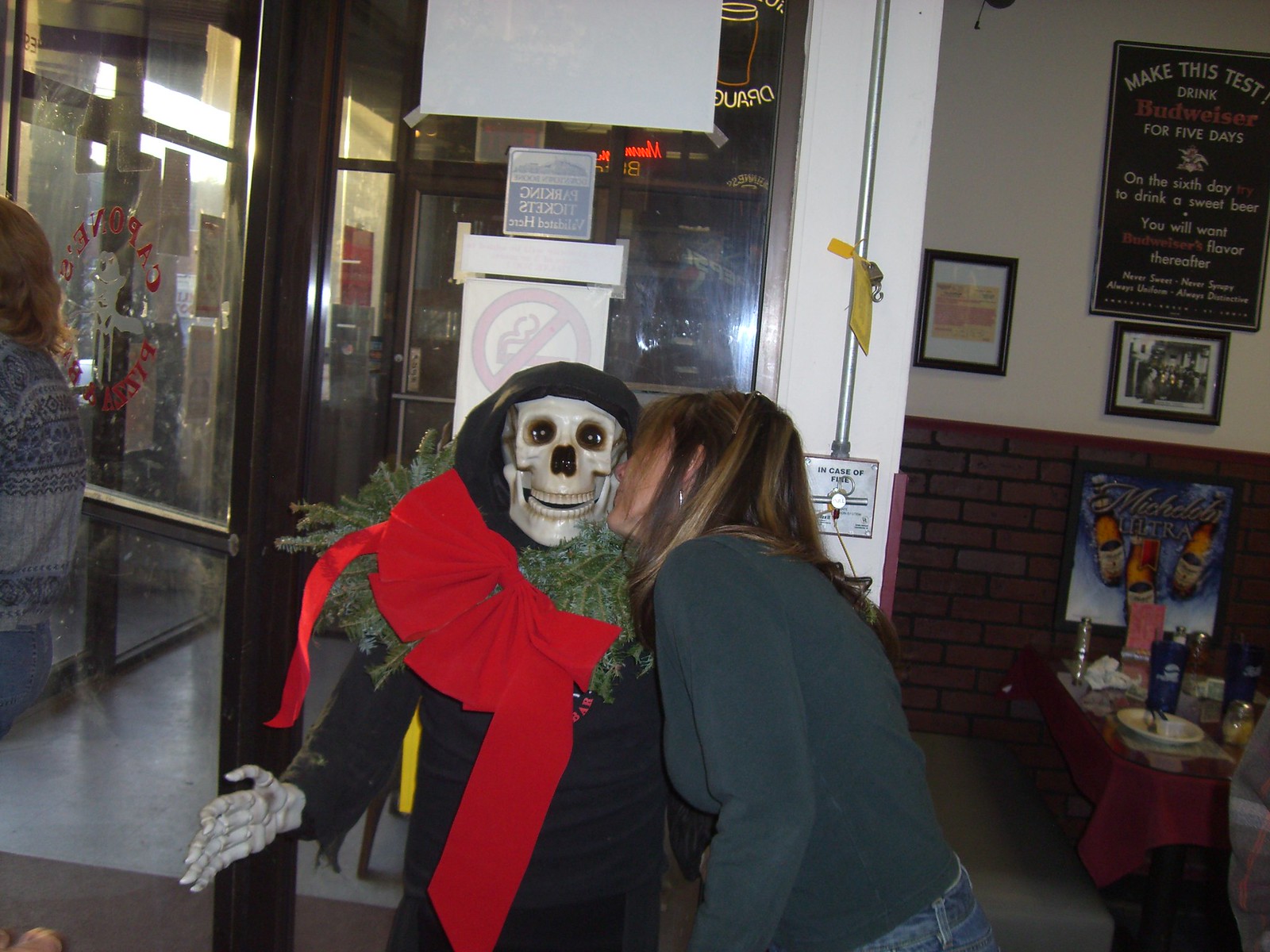In this quirky and detailed photograph taken inside a restaurant, a woman with brown shoulder-length hair, dressed in blue jeans and a blue long-sleeved shirt, is leaning over to kiss the cheek of a Halloween prop: a fake skeleton. The skeleton is dressed in a full black outfit with a black hood, revealing its skeletal face and hand. Adding to the festive decor, it wears a green evergreen wreath around its neck, accented with a large red bow. The skeleton is positioned just inside a window, seemingly in the restaurant's front entryway. To the right of the woman, there's a table cluttered with dirty dishes and glasses, along with a couple of bench seats. Above this setup are pictures and a sign that reads, "Make this test, drink Budweiser for five days. On the sixth day, drink a sweet beer. You will want Budweiser's flavor thereafter." The scene captures a blend of humorous interaction and the casual, slightly cluttered ambiance of the restaurant.